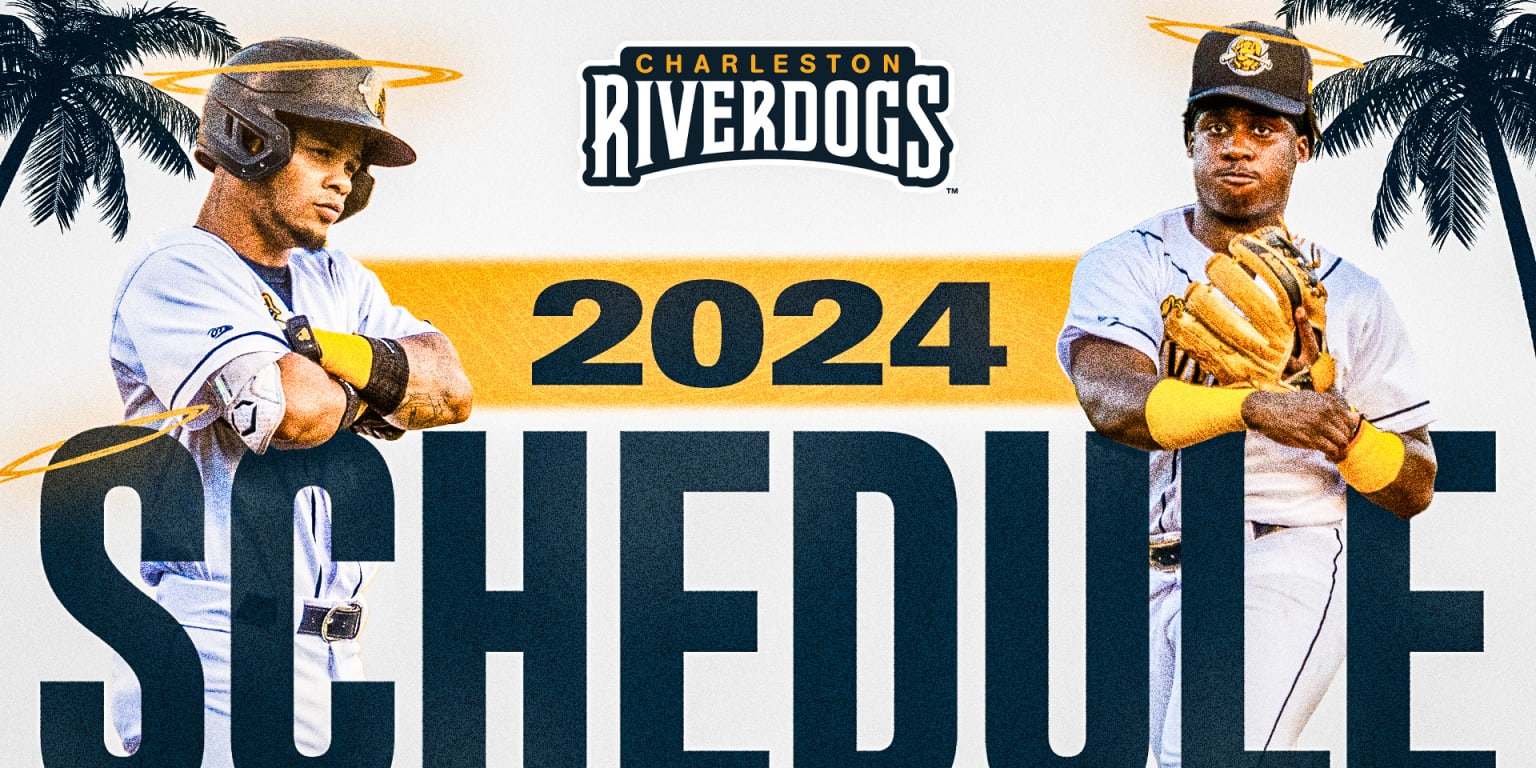The image showcases an advertisement for the Charleston River Dogs' 2024 schedule. At the top, the text "Charleston River Dogs" is displayed, with "Charleston" in small yellow lettering and "River Dogs" in prominent white lettering outlined in dark blue. Below this, "2024 SCHEDULE" is written, with a golden halo adorning the "S" in "SCHEDULE." The background is predominantly white, featuring dark blue-shadowed palm trees on both the left and right edges.

In the foreground, two dark-skinned men in white baseball uniforms with subtle blue or black highlights are prominently featured. The man on the left wears a batting helmet and yellow arm wraps, with his arms crossed in front of him. The man on the right sports a regular baseball cap and a catcher's mitt, looking directly at the camera. Both players have golden halos floating above their heads, adding a unique, almost angelic aspect to the image.